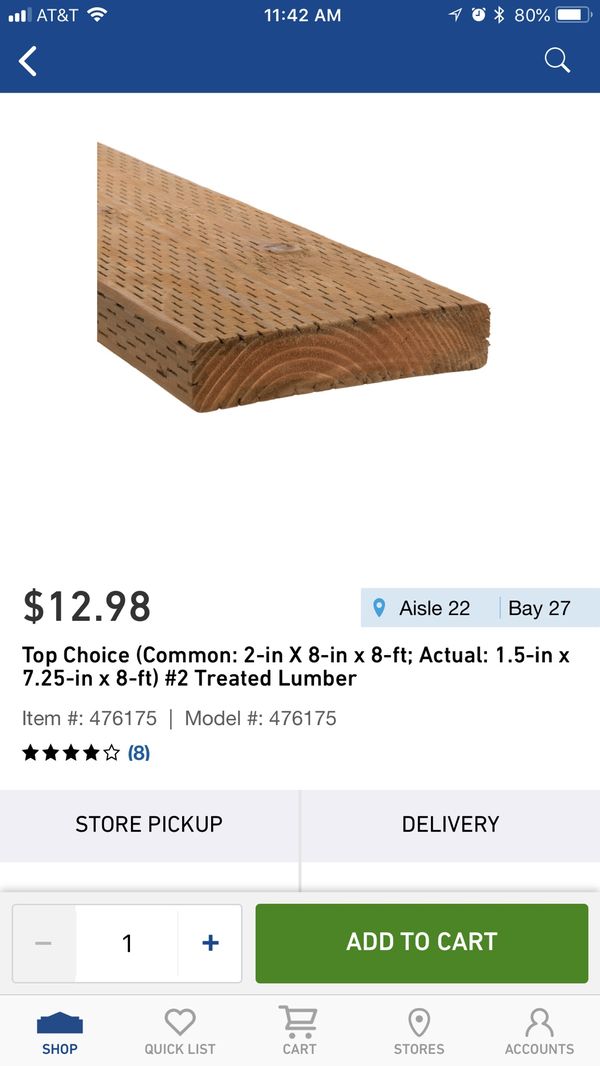This is a detailed screenshot of a smartphone showing a shopping app interface. The top part of the screen features a dark blue border, containing system information: the top right shows full internet signal bars, the AT&T network in white text, a fully filled Wi-Fi icon, and a battery icon indicating 80% charge with the Wi-Fi and alarm icons active. The time, 11:42 p.m., is centered at the top of the screen. A search icon is located under the battery indicator, and a greater than sign appears below the AT&T label.

Below the dark blue top section, the background transitions to white, extending down until about three inches from the bottom. There, an inch-wide light gray strip is followed by a half-inch of white, another inch of light gray, and an inch of white at the bottom. 

In the central section, beneath the header, a piece of brown wood with visible slits and a price tag of $12.98 on the left side is displayed. To the right of the price, there are two blue tabs. The upper tab features a darker blue location icon and text "Aisle 22," while the lower tab reads "Bay 27."

Below the product image, details about the item are provided, including the item number, model number, and a four out of five stars rating. There are two light blue tabs; the left one says "Store Pickup" in black text, and the right one says "Delivery." Underneath these tabs, a quantity selector offers a minus sign on the left and a plus sign on the right, with an "Add to Cart" button in green and white displayed in the center.

At the bottom of the screen, a navigation bar contains several icons: a shop icon with "Shop" below it, a heart icon labeled "Quick List," a cart icon with "Cart" beneath it, a location icon marked "Stores," and an accounts icon with "Accounts" underneath.